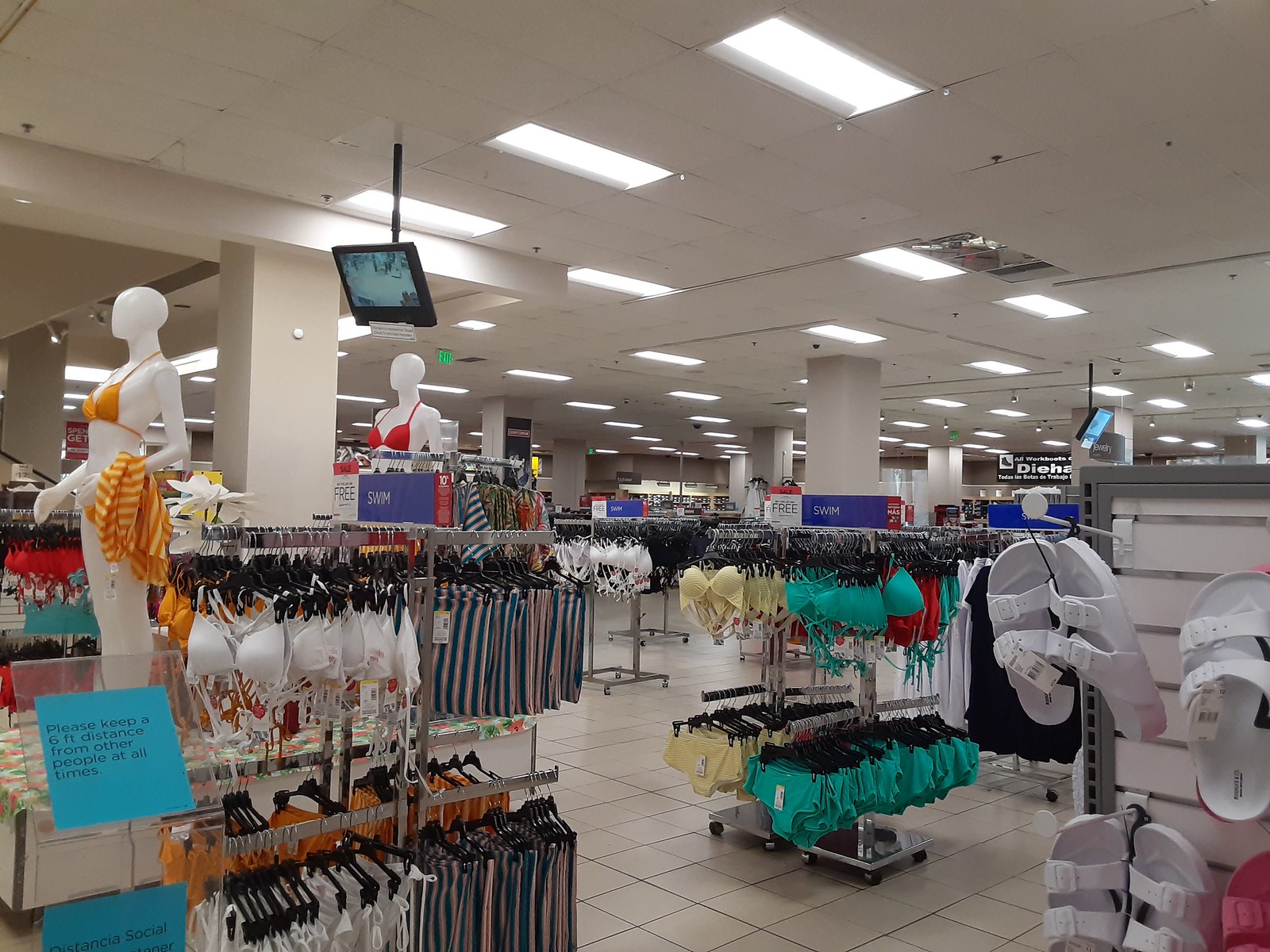This is a detailed photograph of the interior of a women's apparel section within a store. To the right of the image, there is a prominent rack displaying various sandals. On the left side, a collection of bras is organized neatly, adjacent to a display of swimwear. Centered in the image, a standout rack showcases an array of bras in vibrant turquoise and yellow hues, complemented by matching underwear on the lower tier of the same rack. Further into the depth of the store, additional racks filled with a variety of dark and light-colored garments can be seen. Signage reminding customers to maintain a six-foot distance from others suggests proximity to the checkout area. Overhead, standard fluorescent lights are set into conventional ceiling tiles, casting a bright, functional illumination across the scene. The floor beneath consists of 12-inch square brown tiles, adding a warm tone to the store's interior.